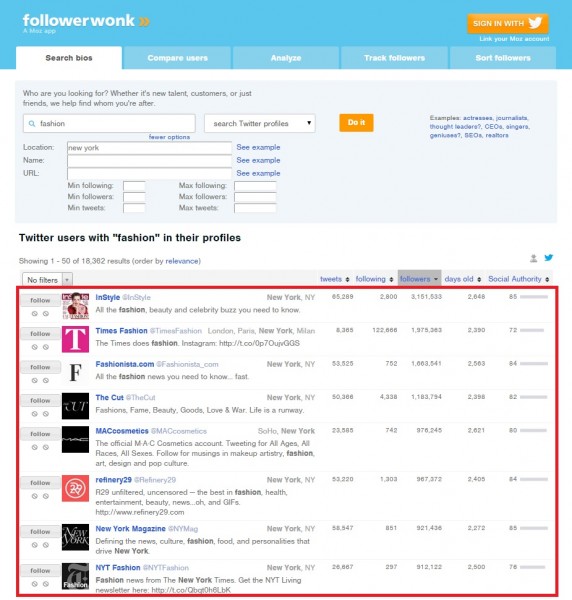This is an image of a webpage for "Follower Walk," featuring a clean, modern interface. The title "Follower Walk" is displayed in bold, lowercase white letters, coupled with a right-pointing arrow. On the right side of the page, there is an option to "Sign in with Twitter," highlighted with the old Twitter logo inside an orange box. Below, a highlighted area features options such as "Search Bios," "Compare Users," "Analyze," "Track Followers," and "Sort Followers."

Underneath these options, a prompt reads, "Who are you looking for? Whether it's new talent, customers, or just friends. We help find who you're after." Adjacent to this, there is a series of boxes, mostly empty except for the first one labeled "Fashion," accompanied by a "Search Twitter Profile" button and an orange "Do it" button.

Near the middle of the page, a section titled "Twitter users with fashion in their profiles" appears. This section features a red-bordered highlighted box with various icons next to it, including a "Follow" button. This layout continues down the page, with each user presented with a picture icon and their name in a consistent format.